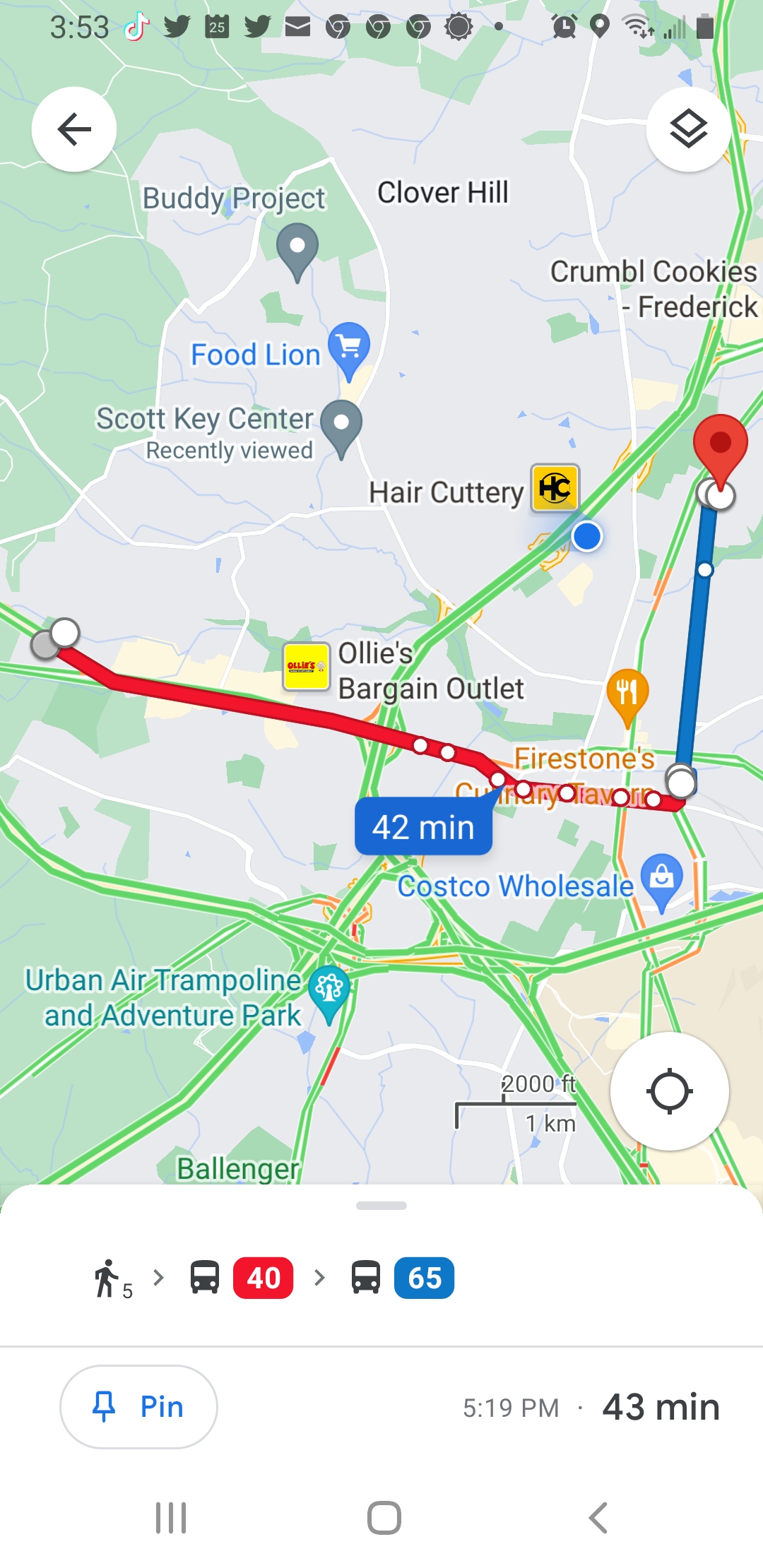This image is a detailed screenshot from the Google Maps application on a Samsung phone, indicated by the home buttons at the bottom. The map is detailing a 42-minute public transportation route, starting with a 5-minute walk, followed by taking the number 40 bus (shown in red) and then transferring to the number 65 bus (shown in blue). The route seems to go through various locations, including a Costco Wholesale, Ollie's Bargain Outlet, and Urban Air Trampoline Adventure Park. Additional landmarks near this route include a Hair Cuttery, Food Lion, Scott Key Center, and a place labeled as Firestones. The map indicates areas such as Clover Hill and near Crumbl Cookies in Frederick. The screenshot was taken at 5:19 PM, capturing all these navigational and locational details.